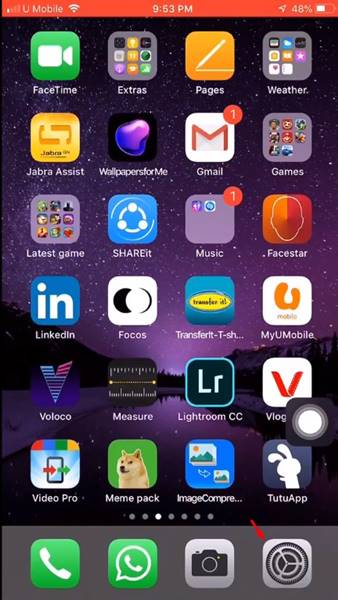Detailed Caption:

Screenshot of a mobile phone likely taken from an Apple device. The status bar at the top indicates connectivity to T-Mobile with a faint Wi-Fi icon on the left side. It shows the current time as 9:55 PM and a battery life at 48% on the right. The background of the screen depicts a serene purple starry sky above black mountains and reflective water. Several app icons are displayed in grid formation. In the upper left corner is the FaceTime app, followed by apps labeled Extras, Pages, Weather, Java, and Assist. The next row features Gmail with one unread message, Games, and Latest Game. Further down, the apps include Music with a notification badge, FaceStar, LinkedIn, Focus, MyLA Mobile, VooHoo, Measure, Lightroom CC, and Vogue. A black-edged button with a white circle partially obscures another icon. Below, the Video Pro, Meme Pack, Image, Compa, and Turn Up apps are visible. Positioned at the bottom of the screen are four prominent icons: a green phone, green WhatsApp, grey camera, and grey settings icon, with a tiny red arrow pointing towards the settings.